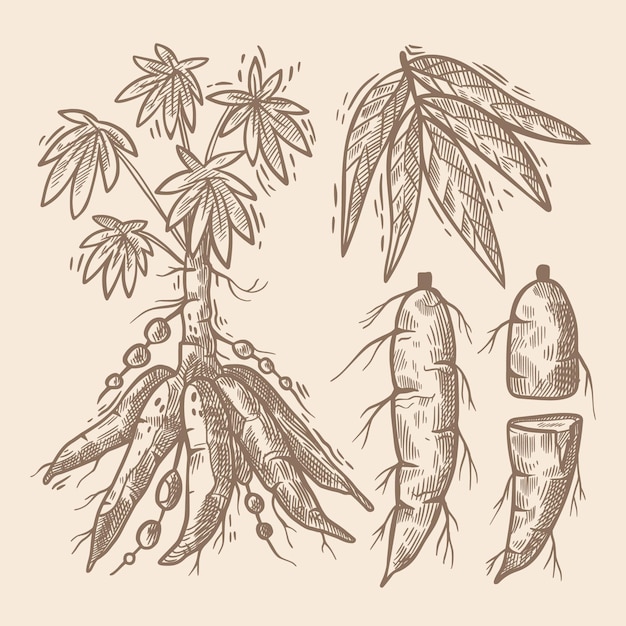This is a detailed drawing, likely sketched on tan or cream-colored paper, showing a plant that appears to have been pulled from the ground. The image primarily focuses on a central plant with roots resembling carrots. From the bottom of the plant, five carrot-like roots extend downward. Attached to the roots is a central stem, which branches out into five pointed, tapered leaves. Additionally, small protrusions or bulbs can be seen on the trunk.

In the upper right corner of the image, there is a close-up section displaying a branch with five pointed leaves. The lower right corner of the drawing showcases one intact carrot-like root, along with another root that has been cut, revealing a separation between its top half and bottom half. The entire illustration is rendered in shades of brown, against a cream or light brown background, and it contains no text. The piece uses monochromatic tones, adding to its detailed and naturalistic appearance.